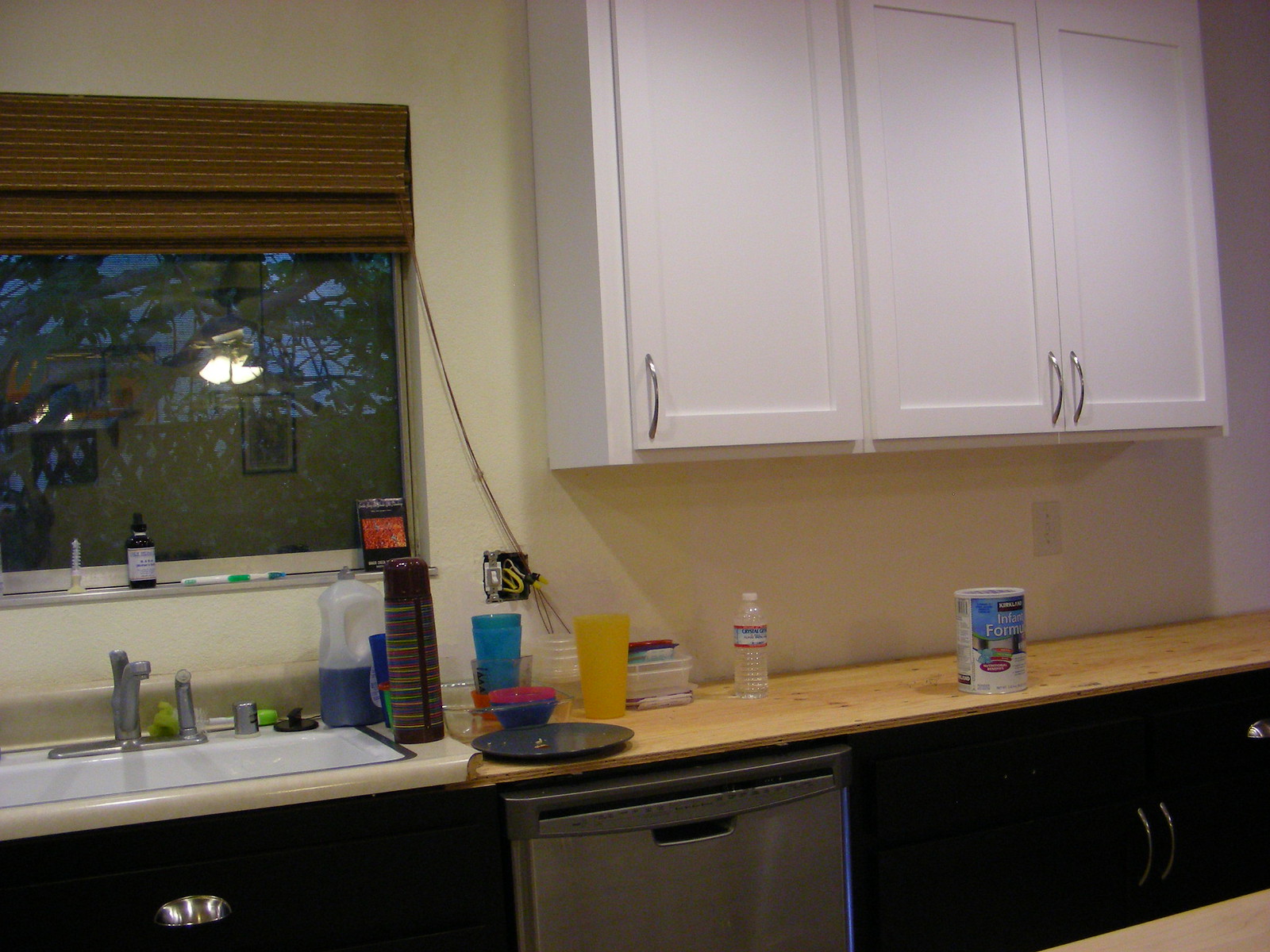This image depicts a kitchen from the perspective of someone standing a few steps away from the sink. 

On the top left, there's a white wall and just below, brown blinds rolled up atop a window. The window itself takes up about half the height of the image and roughly two inches in width. The window frame is white, and on its ledge stands a white object. Next to it sits a small black bottle with a black cap and white labeling. Further to the right, there's a white and green toothbrush with its bristles facing right, and a black package in the corner of the window.

The sink, positioned in front of the window, features a faucet pointed directly at the viewer and a sprayer located to its right. Behind the faucet and sprayer, a green cloth is visible along with a silver soap dispenser, capped. The sink is white with silver trim and sits on a tan countertop.

On the right corner of the countertop, a half-full, blue dishwashing liquid container stands next to a striped coffee mug in shades of green, blue, and brown, with a brown lid. To the right of the mug are some cups and plates, while the brown countertop extends out of the frame on this side. Above, a white shelf descends halfway down the image, continuing out of the frame at the top, and comprising three cabinet doors. The first door's handle is situated in its bottom left corner, while the next door to the right has a handle in its bottom right corner. The third door's handle is also in its bottom left corner.

Below the sink area, there's a black front panel with a drawer that has a silver handle. To its right, there's a silver dishwasher, followed by additional lower cabinets extending out of frame on the right.